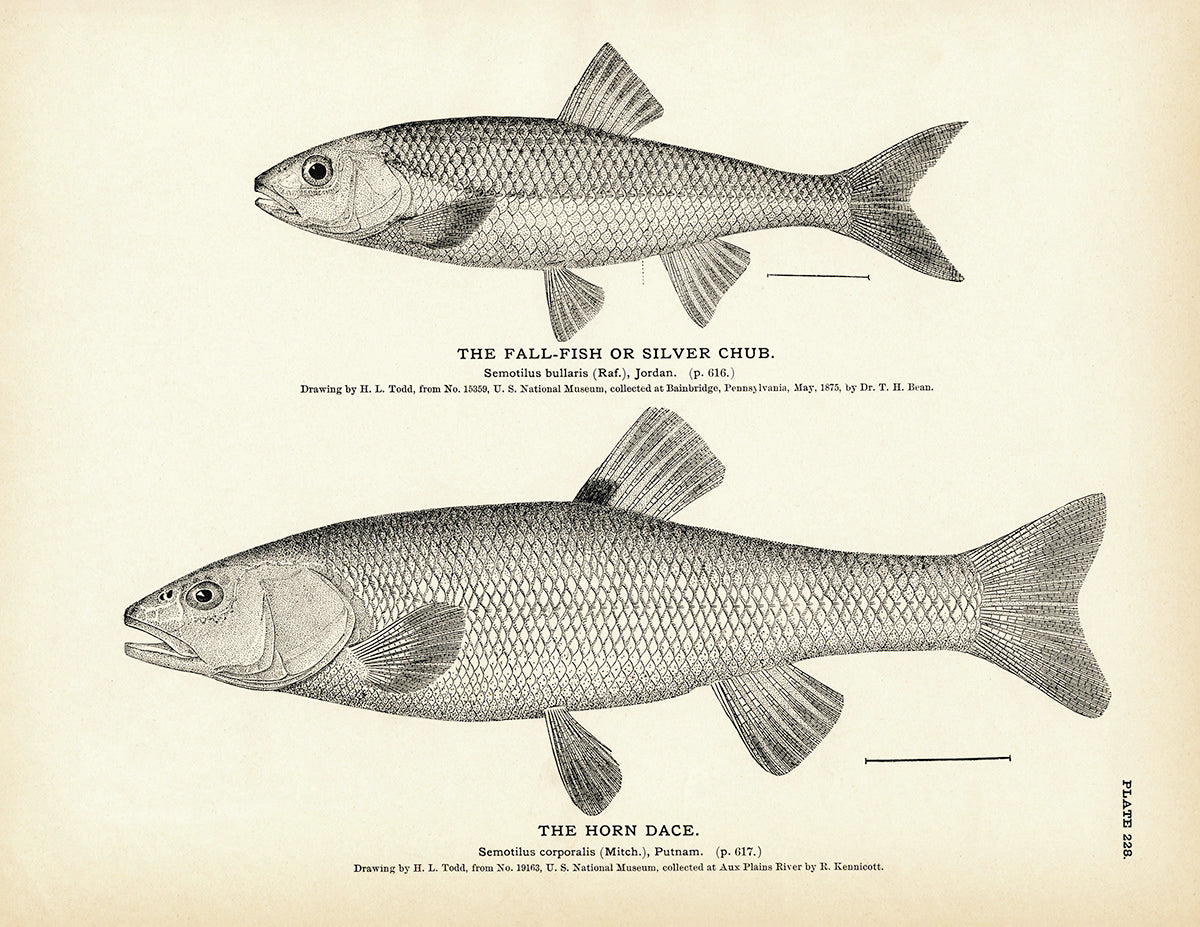This image, sourced from an encyclopedia or an informative book on fish species, features detailed black and white drawings of two types of fish on a yellowed, decaying paper background. The top drawing showcases the "fall fish" or "silver chub" (Semotilus corporalis Mitch., Putnam, p. 617), identified and collected from Bainbridge, Pennsylvania in May 1875 by Dr. T.H. Bean, with the illustration by H.L. Todd. The bottom drawing depicts the "horned dace" (Semotilus corporalis Mitch., Putnam, p. 617), caught at Ox Plains River by R. Kenny Scott, also drawn by H.L. Todd. The paper exhibits a yellowish center transitioning to a brownish-yellow towards the edges, indicating its age and wear. Both illustrations detail the fish from mouth to tail, showing one eye. The fall fish or silver chub is smaller with no distinct markings on its fin, whereas the larger horned dace has a fin with a noticeable black dot. The paper includes small, difficult-to-read text providing additional information about the fish and their collectors.